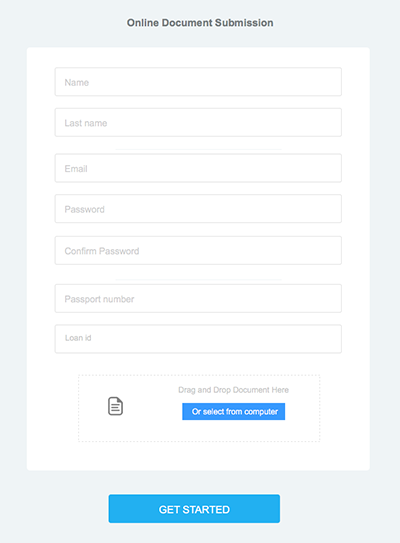The image showcases a screenshot of an online document submission form with a minimalist and straightforward design. The background is light blue, complemented by white form fields that enhance readability. At the top center, the phrase "Online Document Submission" is displayed prominently in bold text, providing a clear purpose for the form.

The form includes several input fields, requesting the user to enter their first name, last name, email, password, confirmed password, passport number, and loan ID. Below these fields is a designated area where users can drag and drop documents for submission.

The design is simple, featuring ample white space that contributes to its clean appearance. At the bottom of the form, there's a bold blue "Get Started" button for users to submit their information.

While the layout is user-friendly and uncluttered, the request for sensitive information such as passport number and loan ID might raise concerns about data security and privacy. The impression given is that the form is functional yet its trustworthiness could be questioned without further context or security assurances.

Overall, the caption outlines the elements of the form clearly while also expressing a degree of skepticism regarding the submission of personal information.